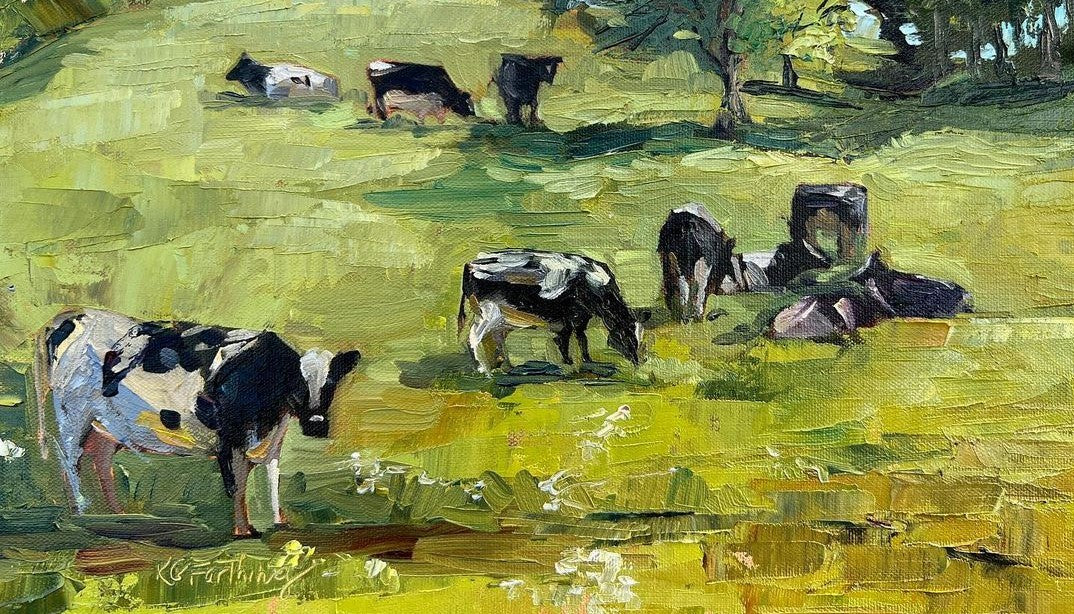This oil-based painting, most likely signed by K. Farthing or K.B. Farthing, vividly captures a pastoral scene with a total of ten cows grazing in a grassy field with various shades of green. The closest and largest cow, situated in the bottom left corner, stands out with its predominantly white body adorned with black spots, a black front, and a distinctive white marking that stretches from the top of its head down to its nose. To the right, in the mid-ground, there's a group of six cows, some of which are grazing while others lay down in the lush grass. In the background, towards the top of the painting, are three more cows, indistinct but visible amidst the textured brushstrokes. Trees punctuate the horizon, with clusters to the center-right and in the top right corner, contributing to the overall pastoral ambiance. The painting's rich texture and visible brushstrokes emphasize its oil-based medium, adding depth and dimension to the serene rural composition. The color palette includes hues of black, white, gray, green, lighter greens, blue, and some brown, enhancing the naturalistic setting.